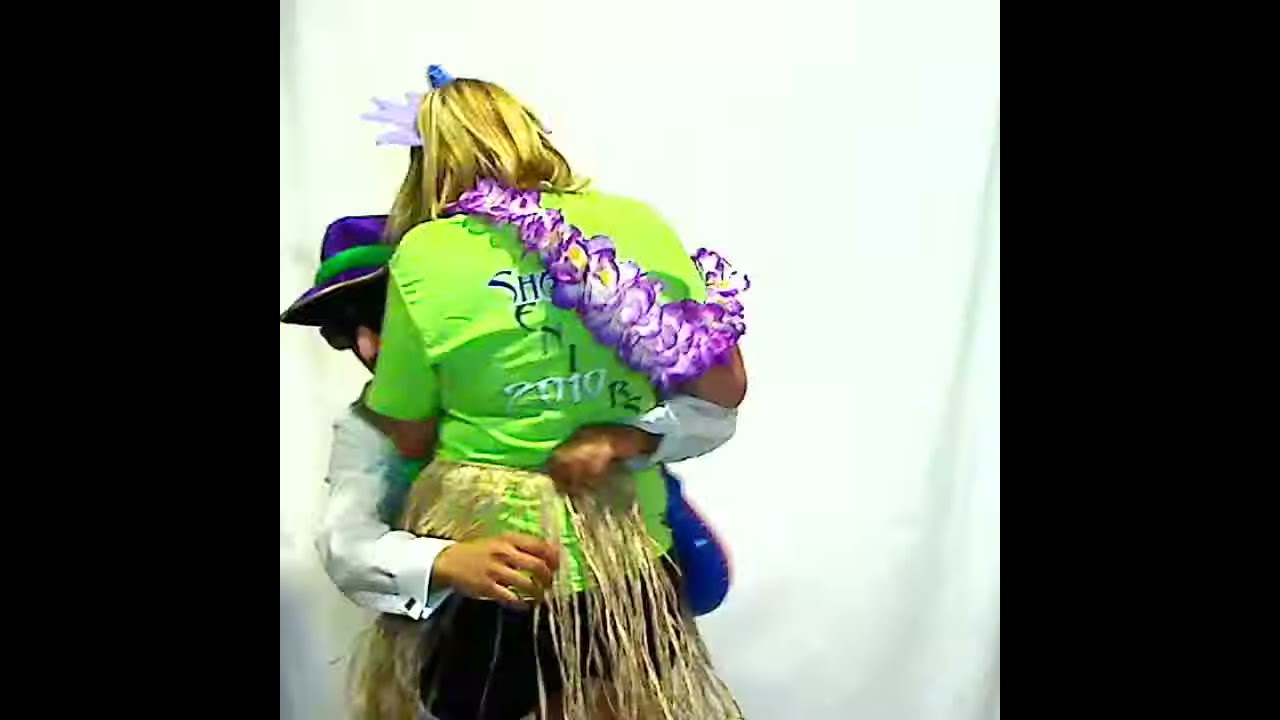In this detailed photograph, we see a woman and a man embracing against a white or cream-colored background. The woman, facing away from the camera, has shoulder-length blonde hair adorned with a small crown-like accessory. She is dressed in a vibrant neon green t-shirt with the words "senior 2010" printed on the back. A tan-colored Hawaiian grass skirt drapes around her waist, completing a festive island look. Over her neck and cascading down her back is a lei made of purple and yellow flowers. Her stance suggests she is standing in front of a shorter man who is sitting or crouching behind her.

The man, whose face is partly obscured by the woman's shoulder-length blonde hair, is wearing a distinctive purple hat with a green band. He sports dark sunglasses and is dressed in a buttoned-up long-sleeved white shirt with decorative cufflinks. His arms are wrapped around the woman’s waist in a tender hug, with his head resting on her chest, peeking over her left arm. This image of shared affection and connection conveys a sense of warmth and intimacy between the two. Black panels can be seen on both sides of the central image, adding a contrasting element to the otherwise light background.